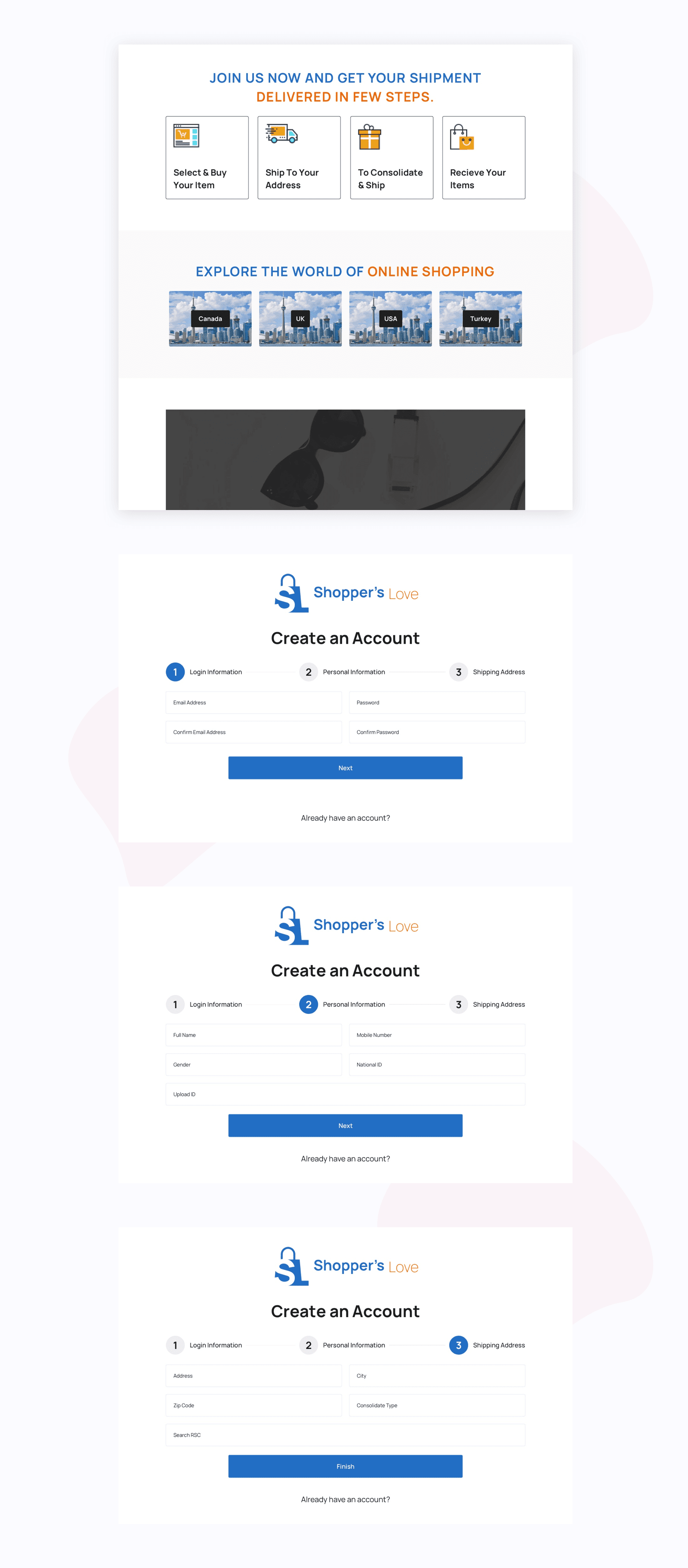The image depicts a multi-section website layout displayed vertically. At the top of the page, a bold headline states, "Join us now and get your shipment delivered in a few steps," accompanied by four horizontally aligned boxes outlining the steps for obtaining a shipment. Below this, a section titled "Explore the World of Online Shopping" features four images, likely of an outdoor mall setting, with a prominent black sign and cloud-filled sky in the background.

Continuing down, there's a large vertical box showcasing a pair of sunglasses, set against an ambiguous background that might be a towel or some other indistinct object. Further down, the page prompts users with the phrase "Shoppers Love" and directs them to "Create an Account," providing a form and a blue clickable bar for submission. This layout repeats twice more, each with an identical format but designated as "Step 1," "Step 2," and "Step 3," indicated by blue circles, guiding the user through a step-by-step account creation process.